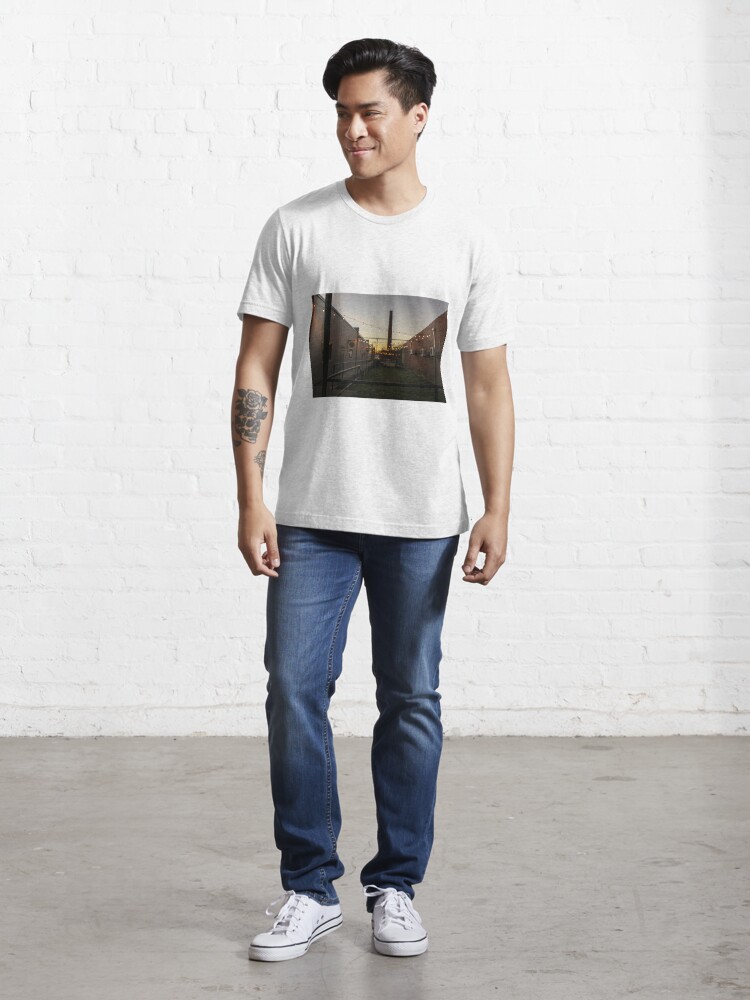The image is a color portrait photograph of a young man in his 20s, modeling casual clothing. He stands at the center of the vertically aligned rectangular frame on a gray concrete floor, against a backdrop of a white-painted brick wall. The man has short, styled black hair and a tattoo on his right forearm, which depicts a flower atop a skull. He is partially smiling, looking off to his right, and exudes a joyous, amused expression.

He is dressed in a white crew-neck T-shirt with a short sleeve, featuring a rectangular graphic of an urban alley scene with buildings flanking a central element that appears to be a smokestack or sunset. He pairs the shirt with blue jeans and white sneakers, which have a gray stripe at the sole. Both his hands hang naturally by his sides. The photograph captures a moment of casual, realistic fashion in a seemingly urban setting.